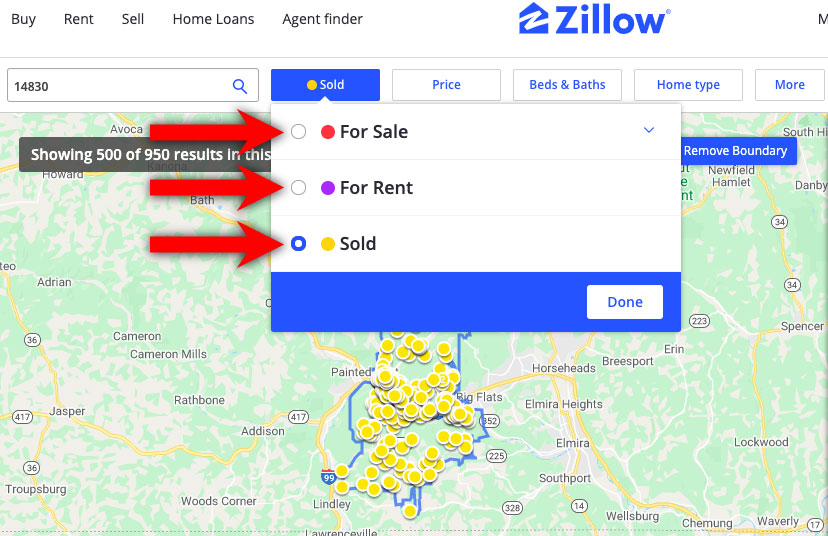A Zillow map interface for purchasing a home is depicted in this image. At the top of the screen, the Zillow logo is prominently displayed in blue, accompanied by navigation options to the left labeled "Buy," "Rent," "Sell," "Home Loans," and "Agent Finder." In this particular instance, a ZIP code, "14830," has been entered into the search bar. Beneath the search bar, three main options are displayed for filtering properties: "For Sale," "For Rent," and "Sold," each indicated by a distinct red arrow. The user has selected the "Sold" filter, which is highlighted and confirmed by a "Done" button.

In the background, the map is populated with numerous yellow dots, each representing a sold property. The map also uses blue dots to indicate rental listings and red dots for properties that are currently for sale. The towns visible on the map include Lawrenceville, Lindley, Big Flats, Painted Post, Horseheads, Elmira, and Elmira Heights.

Additional filters are available for customization, such as price range, number of beds and baths, home type, and more. The user can expand their search area by choosing to remove boundary restrictions. Notably, the interface indicates that it is displaying 500 of the 950 available results.